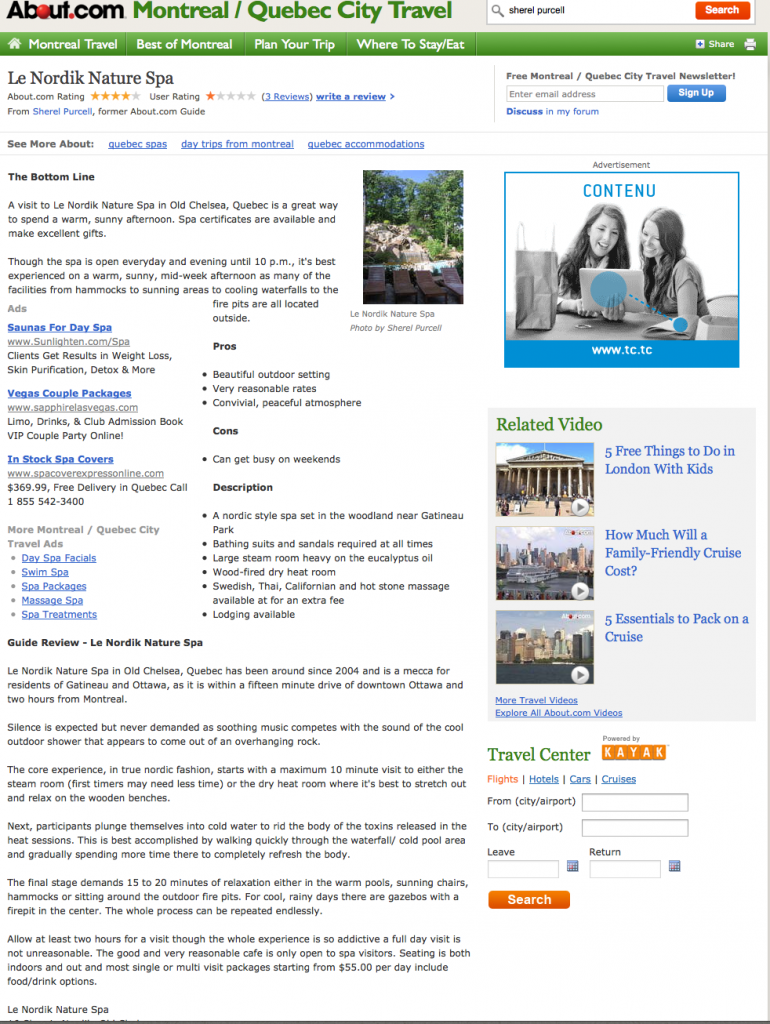This image is a screenshot from the now-defunct website, about.com, likely dating back several years. In the upper left-hand corner of the header, the about.com logo is prominently displayed in bold black font, with the letter "O" depicted as a red circle. Adjacent to the logo, the green text reads "Montreal/Quebec City Travel."

Beneath the header, in the same shade of green, the navigational menu features white fonts that direct users to sections such as "Montreal Travel," "Best of Montreal," "Plan Your Trip," and "Where to Stay/Eat." Further down, there's a notable listing for the "Nordic Nature Spa," which boasts a four out of five-star rating. The clarity of the font in this section is somewhat difficult to discern, but a headline titled "The Bottom Line" is visible, followed by a brief description.

On the right side of the webpage, a vertical navigational menu appears. At the very top, there's a black and white advertisement featuring two white women seated at a table and looking at a laptop. Directly below the ad, a headline "Related Video" precedes three thumbnail images of videos. The first image appears to be a parliament-type building, the second is a panoramic view of a city from a harbor perspective, and the third image is a similar cityscape view.